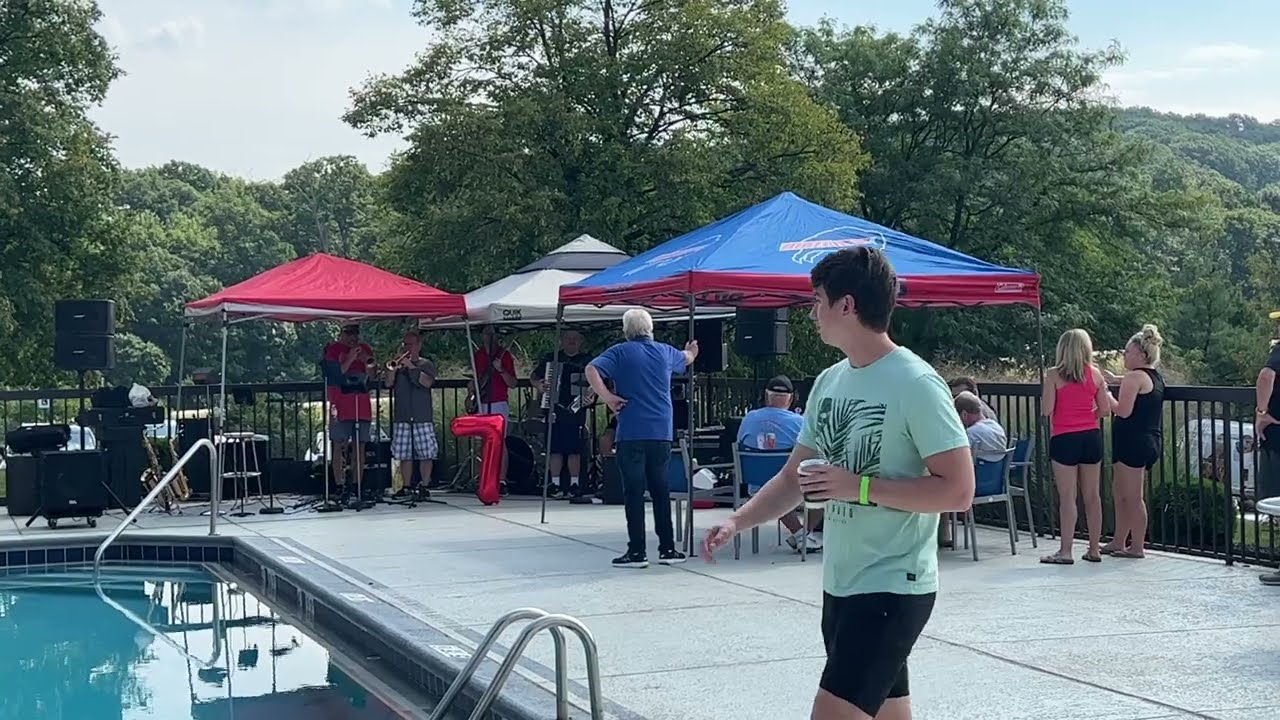The image depicts a lively outdoor poolside party. In the foreground, a teenager wearing a light green shirt, black pants, and a green wristband holds a drink in his left hand. To his left is a pool with chlorine-tinted water and visible ladders and steps. Surrounding the pool area, several people are gathered, some sitting in blue chairs on a deck and others conversing under various canopies. Notably, a Buffalo Bills canopy stands out, accompanied by other canopies with red and white tops. 

Behind the canopies, a lush backdrop of tall green trees, resembling a forest, can be seen against a partly cloudy blue sky. Under the white and red canopies, a live band is performing, featuring musicians playing brass instruments, a guitar, and an accordion. A blow-up number seven is positioned in front of the band. The festive setting suggests a midday event, adding to the vibrant and dynamic atmosphere of this poolside gathering.